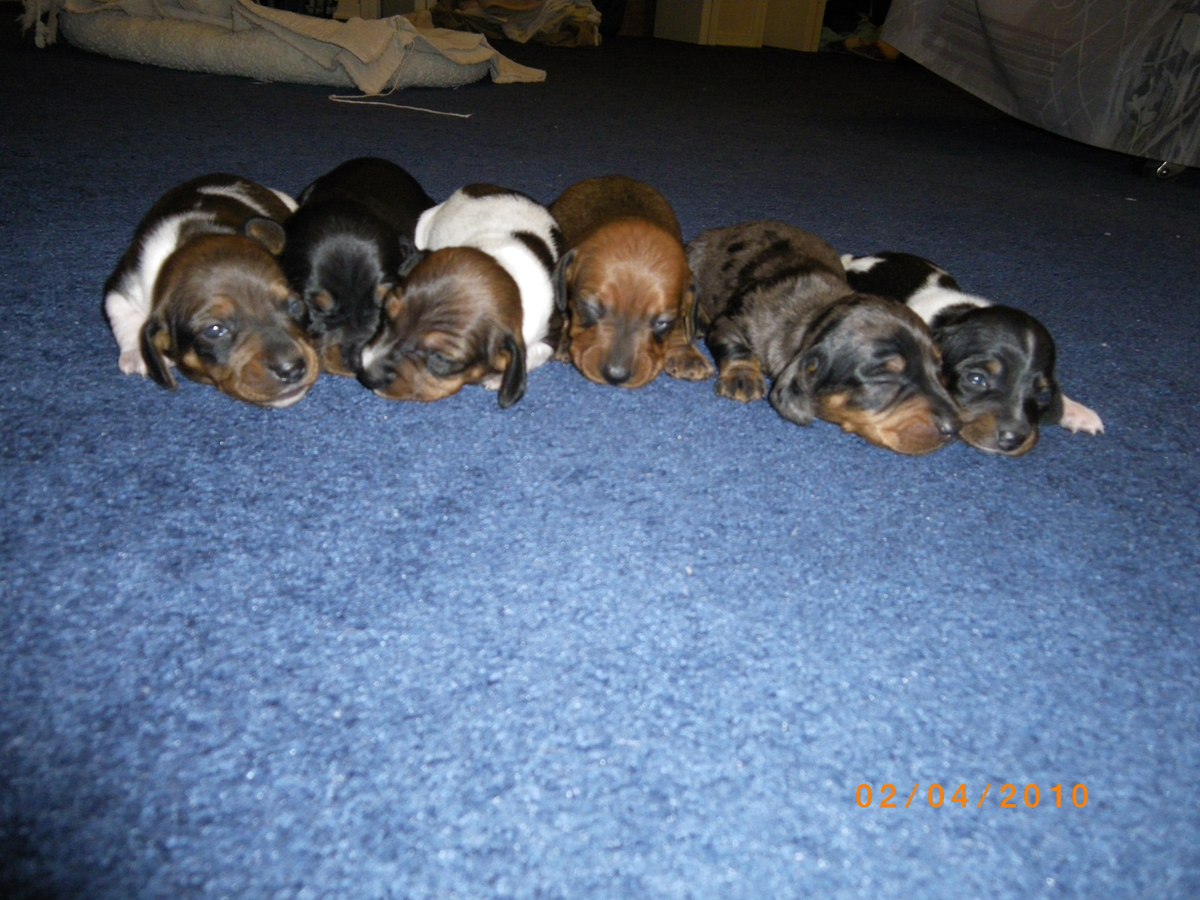This indoor color photograph captures a heartwarming scene of six adorable, very young puppies, all of the same breed, arranged in a cozy, close-knit alignment on a light blue carpet. They are positioned towards the upper portion of the image, each pup facing the camera with varying facial expressions of sleepiness or curiosity. The backdrop features a blue blanket and what appears to be a dog bed or an air mattress in white, adding to the homely ambiance.

From left to right, the first puppy has a medium brown head and a black and white body, with its eyes open. The second puppy, entirely black, is peacefully sleeping. The third puppy, mostly white with some large brown spots and a brown head, also appears to be asleep. At the center, a rust-colored brown puppy with slightly darker eyes lays serenely. To this central pup's right, the fifth puppy has a brown muzzle with a black or dark gray body, and like the first, its eyes are open, taking in the environment. Finally, the sixth puppy, characterized by its black head, black and white body, and distinctive white left paw stretching forward, completes the lineup. This pup also has light brown eyebrows and mouth surroundings.

A pale red or orange text overlay in the lower right corner of the photo marks the date as 02-04-2010, with no other text present. This image beautifully encapsulates a moment of early puppyhood, blending both tranquility and curiosity.